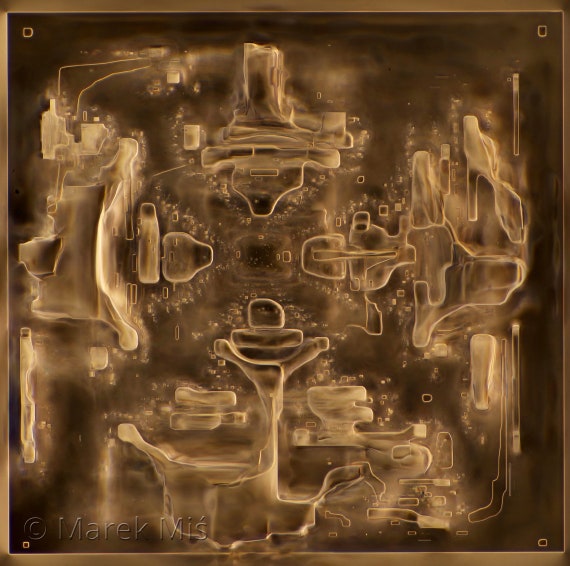This is an abstract painting by the artist Marque Marěk Míš, as indicated by the signature in the bottom left corner. The artwork features a predominantly brown color palette, ranging from very pale, almost white cream shades to dark, almost black tones. The hues also include metallic, brassy, and coppery tints, giving the piece an overall tarnished brass appearance. The painting has a complex and intriguing design with a mixture of curving, warping textures and more structured, squared-off shapes with rounded corners. These shapes are arranged in a pattern that creates an almost mirrored or mandala-like effect, radiating from a central focal point and giving the impression of looking down a hallway. The composition suggests a flowing, interconnected system, akin to a loose, floating circuit board. The entire piece is framed in brown, enhancing the sense of cohesion within the varied brown shades of the painting.